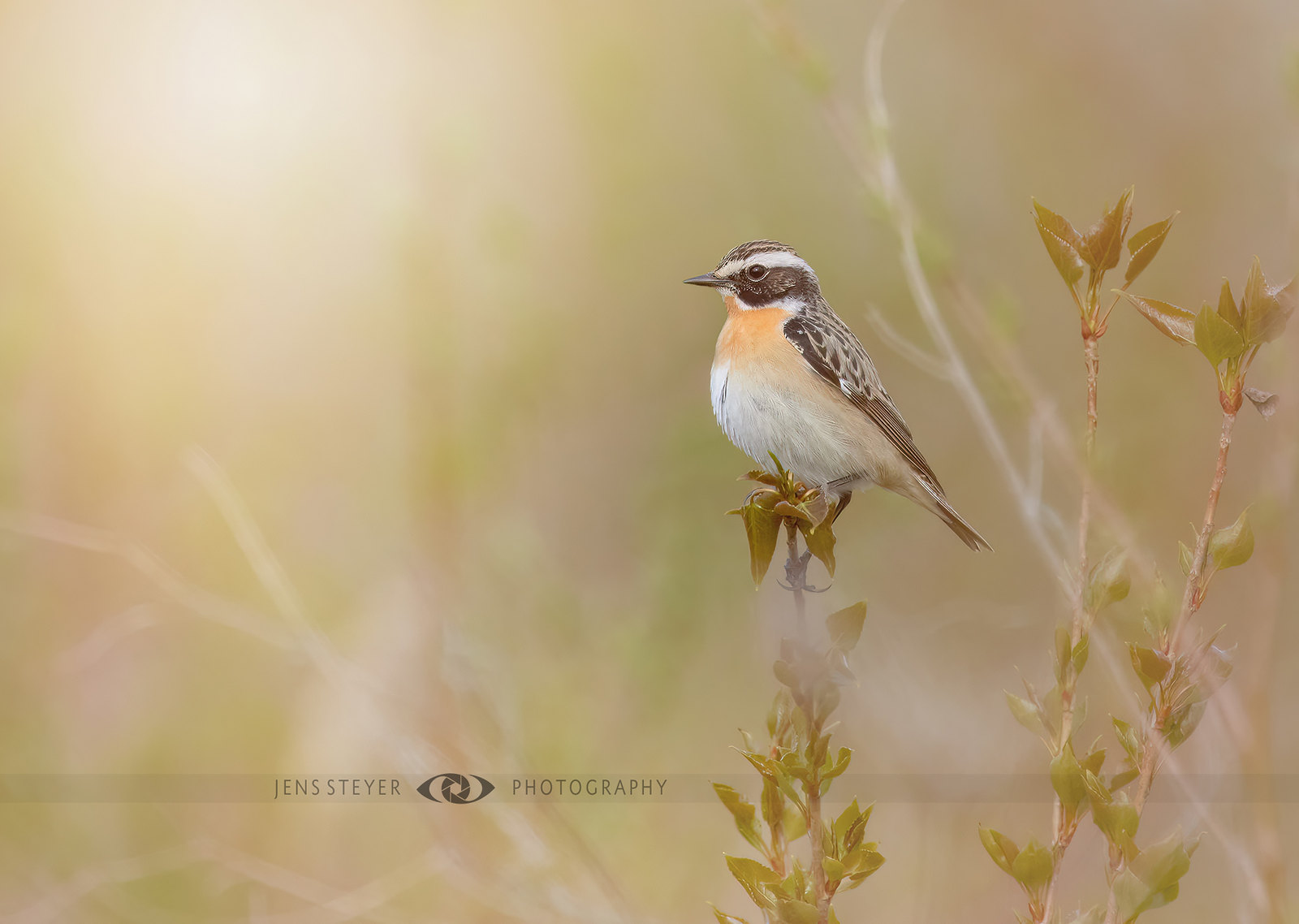This detailed color photograph depicts a small bird perched on a slender, leafy plant branch. The bird is mostly brown with white streaks, and its underbody is predominantly white. It also has an orange hue near its neck and a distinctive white line running from its beak down its back. The bird is shown in a side profile, facing to the left, with its brown beak clearly visible. Surrounding the bird are several similar plants with green leaves, and the background is a soft blur of green and brown tones, enhancing the focus on the bird. The overall atmosphere suggests it is daytime, and the vivid colors highlight that it is captured in the wild. At the bottom of the photograph, a watermark reads "Jens Stier Photography" alongside a logo, indicating this is a professional photograph.